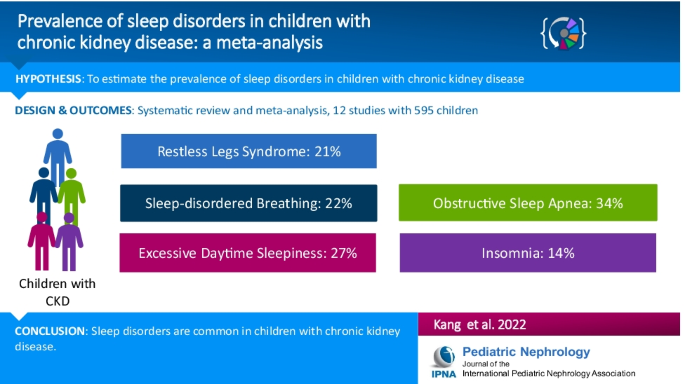This image is a detailed color diagram illustrating the prevalence of sleep disorders in children with chronic kidney disease (CKD), based on a systematic review and meta-analysis involving 12 studies with 595 children. The predominant colors in the diagram include various shades of blue, green, purple, dark magenta, and pink. 

At the top, the title is prominently displayed in blue: "Prevalence of Sleep Disorders in Children with Chronic Kidney Disease: A Meta-Analysis." Below this, in light blue, is the hypothesis: "To estimate the prevalence of sleep disorders in children with chronic kidney disease."

Further down, the background turns white where the "Design and Outcomes" section details the systematic review and meta-analysis. This segment emphasizes the findings from 12 studies, detailing the prevalence of specific sleep disorders among the children surveyed:

- Restless Leg Syndrome: 21% (highlighted in blue)
- Sleep Disordered Breathing: 22% (highlighted in dark blue)
- Excessive Daytime Sleepiness: 27% (highlighted in pink)
- Obstructive Sleep Apnea: 34% (highlighted in green)
- Insomnia: 14% (highlighted in purple)

On the left side of the diagram, five figures of children are shown in blue, dark blue, grey, pink, and purple, labeled as "Children with CKD." The right side specifies that the data pertains to children with chronic kidney disease (CKD).

At the bottom left, the conclusion reads, "Sleep disorders are common in children with chronic kidney disease." The image credits "Kang et al., 2022," and it is published in the "Journal of the International Pediatric Nephrology Association" (IPNA).

Additionally, the diagram features the publication's affiliation and the year: CAM-ADAPT 2022.